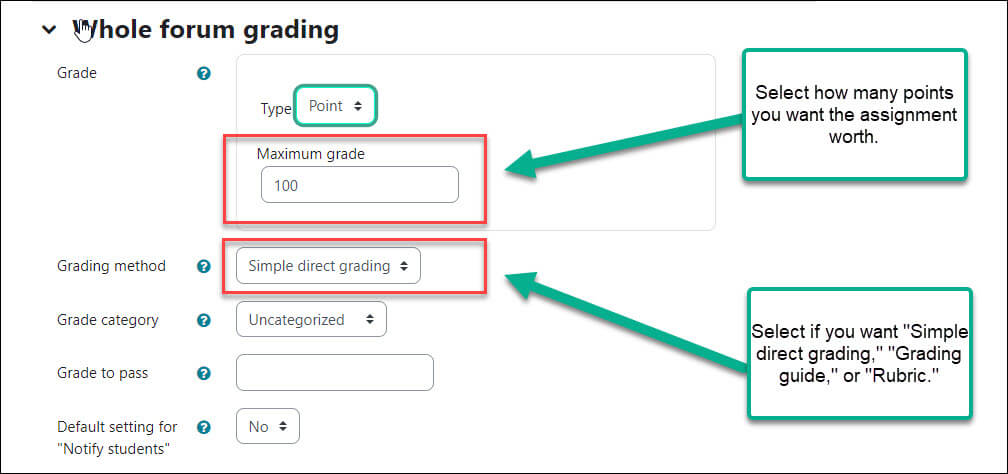To the left, there is a small arrow pointing downward labeled "Whole Forum Grading." Below it, the word "Grade" is followed by a question mark, indicating uncertainty or a prompt for input regarding the grading method. Following this are prompts for "Grade Category," "Grade to Pass," and "Default Setting for Notify Students" (the latter enclosed in quotations). The word "Type" is displayed next to a green rectangle labeled "Point."

Enclosed within red lines, the text "Maximum Grade" displays a value of "100." Adjacent to this, a green box with an arrow points to the text, "Select how many points you want the assignment worth."

In an additional red box with outlined text, the term "Simple Direct Grading" is visible. To the right, a green arrow points to a selection for the grading method, offering options for "Simple Direct Grading," "Grading Guide," or "Rubric."

Further to the right, there is a category labeled "Uncategorized" accompanied by an empty text box. Finally, beside the "Default Setting for Notify Students" prompt, the word "No" is displayed.